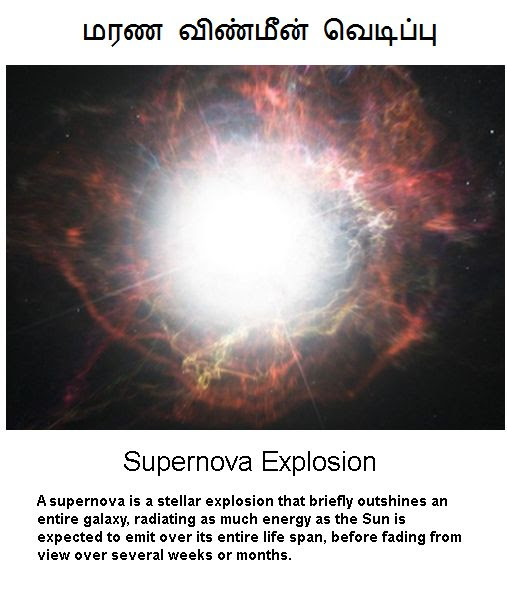The image depicts a breathtaking supernova explosion set against a deep black background. At the core of this cosmic spectacle is an intensely bright white light, surrounded by an eruption of vibrant red, orange, and yellow hues that extend outward like lightning bolts. These vivid colors intermingle with hints of purple and blue, creating a dynamic and mesmerizing display that radiates outward in a circular pattern before gradually fading into the surrounding darkness. On the top and outer edges of the image, there are symbols and text in a language that appears to be Hindi, while the bottom part features a bold, sans-serif English caption that reads: "A supernova is a stellar explosion that briefly outshines an entire galaxy, radiating as much energy as the Sun is expected to emit over its entire lifespan before fading from view over several weeks or months." Scattered across the top right corner are small white dots resembling distant stars, enhancing the celestial ambiance of this outer space phenomenon.